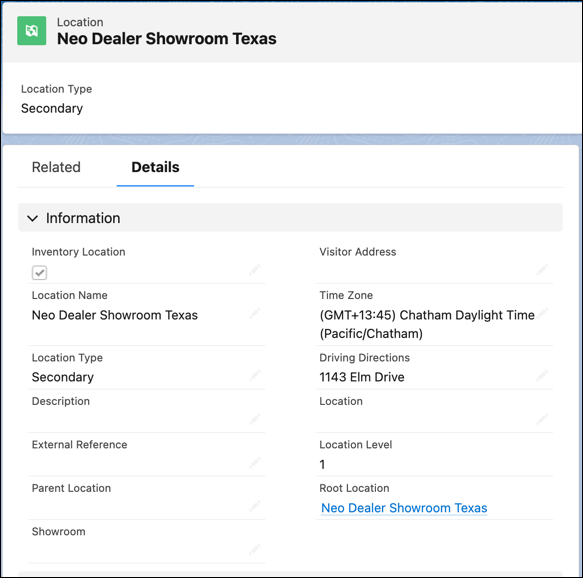The image displays detailed information about the location of a Neo-Dealer showroom in Texas. At the upper left corner, a small green square logo featuring a wavy white rectangle is visible. Adjacent to it, text reads "Location: Neo-Dealer Showroom, Texas." Directly below, it indicates that the location type is "Secondary." 

The interface includes two tabs, "Related" and "Details," with the "Details" tab highlighted. Within this tab, a dropdown menu exposes further specifics: the inventory location, the showroom's name "Neo-Dealer Showroom, Texas," and reiterates the location type as "Secondary." Some categories remain unfilled.

Additional information includes the time zone, specified as Chatham Daylight Time, and the address for driving directions, 1143 Elm Drive. The location level is identified as 1, and a blue hyperlink labelled "Neo-Dealer Showroom, Texas" is indicated as the route location.